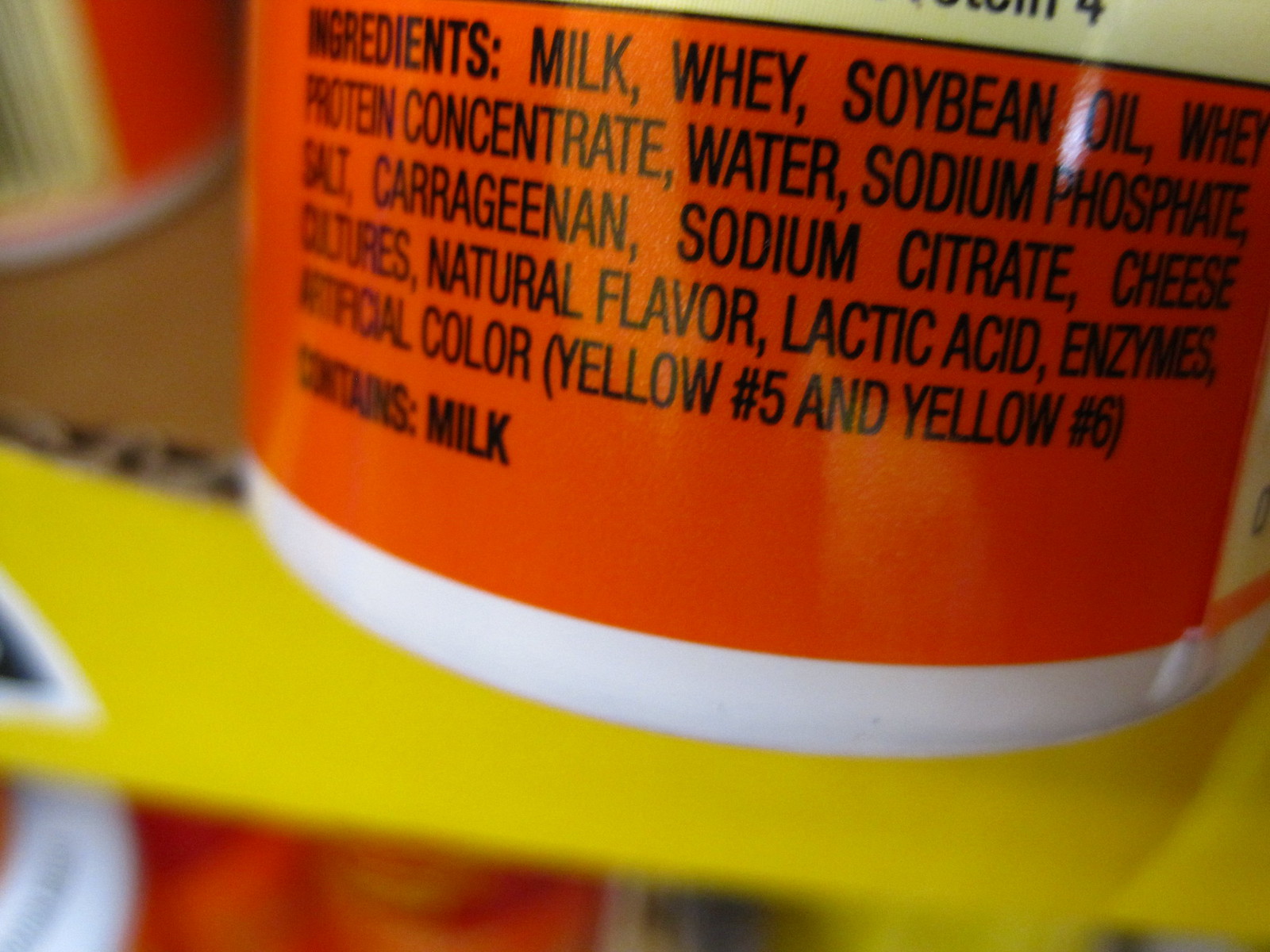This photograph captures a close-up of a product label on a yellow shelf, showcasing the ingredients of a bottled item. The label, prominently orange and white, lists the ingredients in black font: milk, whey, soybean oil, whey protein concentrate, water, sodium phosphate, salt, carrageenan, sodium citrate, cheese cultures, natural flavor, lactic acid, enzymes, artificial flavor, Yellow 5, and Yellow 6. Additionally, a bold statement indicates the product contains milk. The background reveals a partial view of another identical bottle with the same orange and white label. Just below, the tops of several orange bottle lids are visible, enhancing the color scheme of the scene.